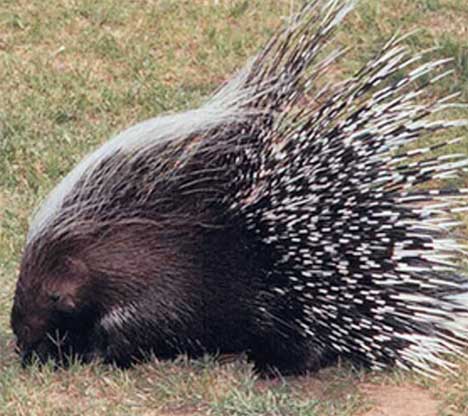In this image, a dark brown porcupine is positioned centrally on a patch of freshly cut green grass, with light brown dirt faintly visible underneath. The porcupine has distinctive black eyes and a body covered in long, white fur that starts from the back of its head, forming a striking mohawk-like strip, and cascades backward. Its characteristic quills, which are black with white tips and dotted patterns, flare outward in a defensive display, resembling a splayed peacock's tail. The porcupine's quills suggest it might be in a defensive posture. The background features muted tones of greens and yellows. The porcupine appears to be either eating the grass or curiously looking down at it.